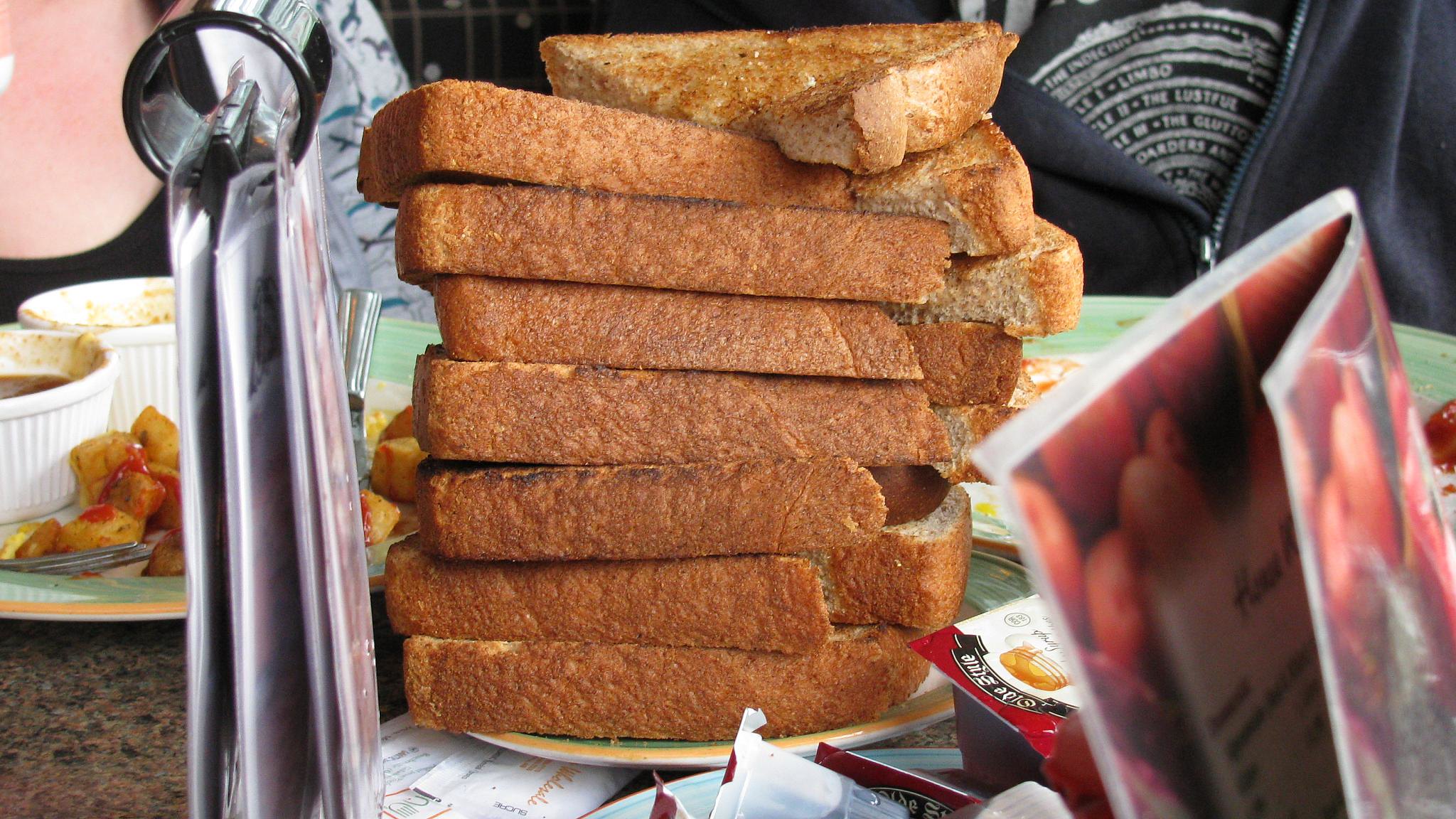The photograph, taken in color and landscape format, captures a bustling breakfast scene at what appears to be a restaurant. Dominating the center of the image is a towering stack of toast, cut diagonally and composed of about 16 slices arranged in two layers. The toast is light brown, almost resembling French toast. To the immediate right of this stack lies a folded menu, partially obscuring what appear to be honey or jam packets. Moving further left, there's a partially eaten plate featuring diced potatoes, possibly hash browns drizzled with ketchup, and accompanied by two small ramekin cups, presumably containing some kind of dipping sauce.

In the background, partially obscured but present, are two people engaged in conversation. The person on the right, wearing a dark navy blue hoodie and a black shirt with the text "Limbo" visible, sits next to a woman on the left, dressed in a white and blue patterned jacket over a black top. The image suggests a cozy, albeit cluttered, breakfast setting with a variety of meal components peeking through, reflecting the lively atmosphere of a busy restaurant morning.